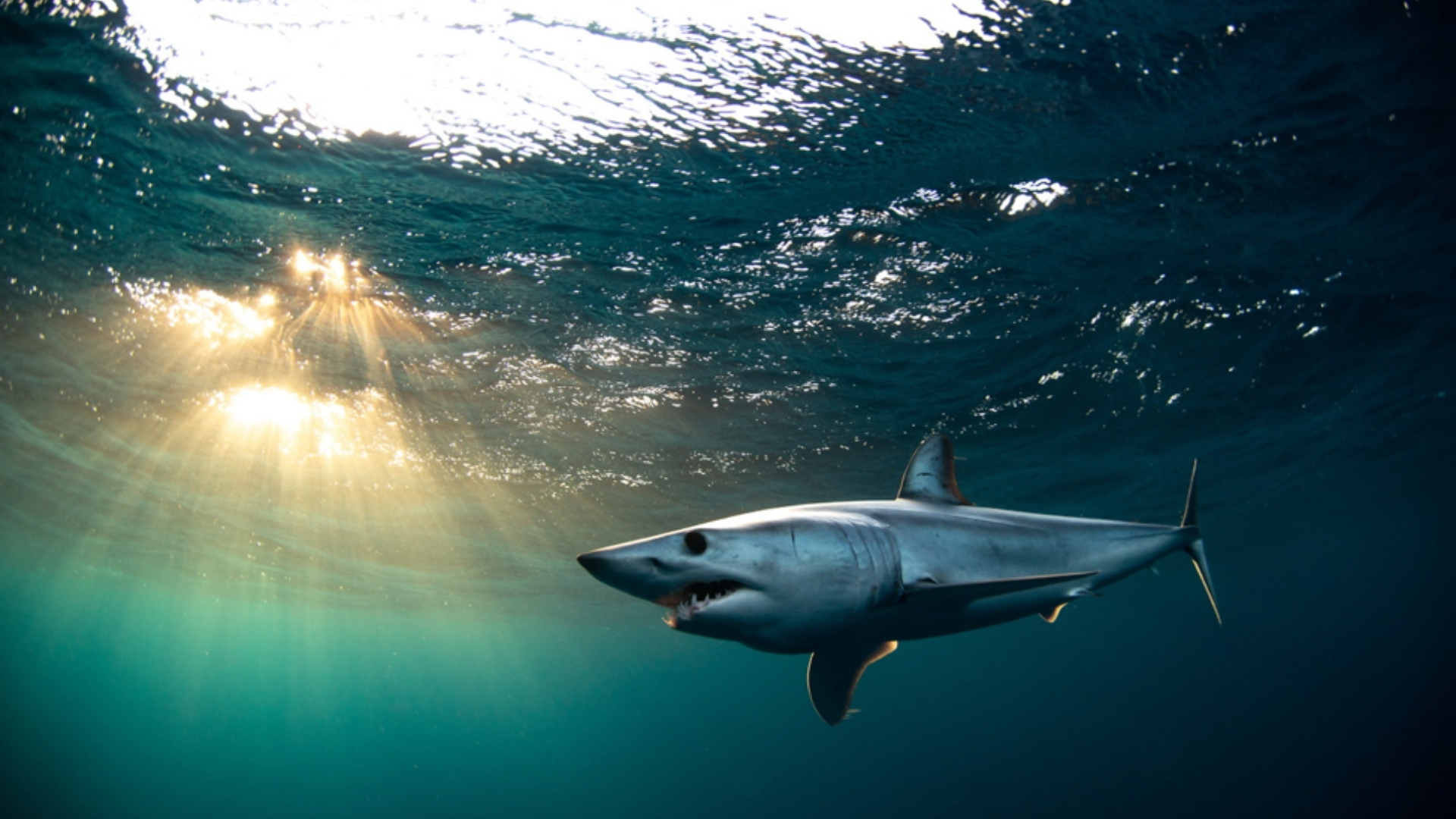This image depicts a silver-hued shark swimming in the deep, greenish-blue water. The shark, positioned in the lower right corner of the frame, is angled towards the bottom left, showcasing its sleek profile with a pointed nose, a visible black eye, several gill slits, sharp teeth within its slightly open mouth, and clearly defined pectoral, dorsal, and tail fins. The water around the shark transitions from darker tones on the right to a lighter greenish-blue color on the left, where sunbeams pierce through the surface, casting a yellowish light that illuminates the top of the shark and creates reflections on its body. Above, the surface of the water is visible, highlighted by a bright white section that contrasts with the underwater blues. The overall scene evokes a sense of motion and light interplay in an underwater realm.